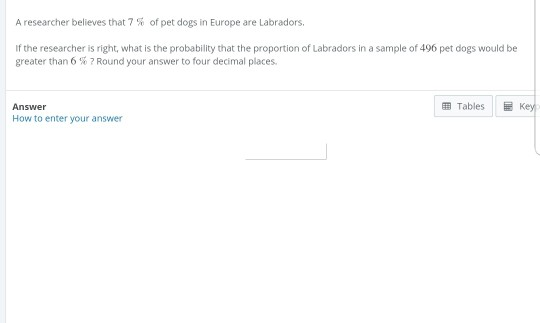This screenshot captures part of an online quiz focused on a probability problem. The image has a white background. On the left side, there's a thin, vertical, grayish bar. Another thin, grayish line curves off to the right at the bottom, forming an almost hook-like shape.

Centered in the image is a rectangular, landscape-style text box containing an instructional math problem. The text reads: "A researcher believes that 7% of pet dogs in Europe are Labradors. If the researcher is right, what is the probability that the proportion of Labradors in a sample of 496 pet dogs will be greater than 6%? Round your answer to four decimal places." Notably, the word "Labrador" is capitalized.

Below this problem, a very thin gray line extends horizontally from the left to the right sides of the image. On the lower-left side, there is black text that reads "Answer," directly below which is blue text stating "How to enter your answer." On the lower-right side, there are two gray buttons: the first labeled "Tables" with an icon of a table, and the second labeled "Keypad" with an icon of a keypad. Additionally, a sideways L-shaped element is visible at the bottom center of the image.